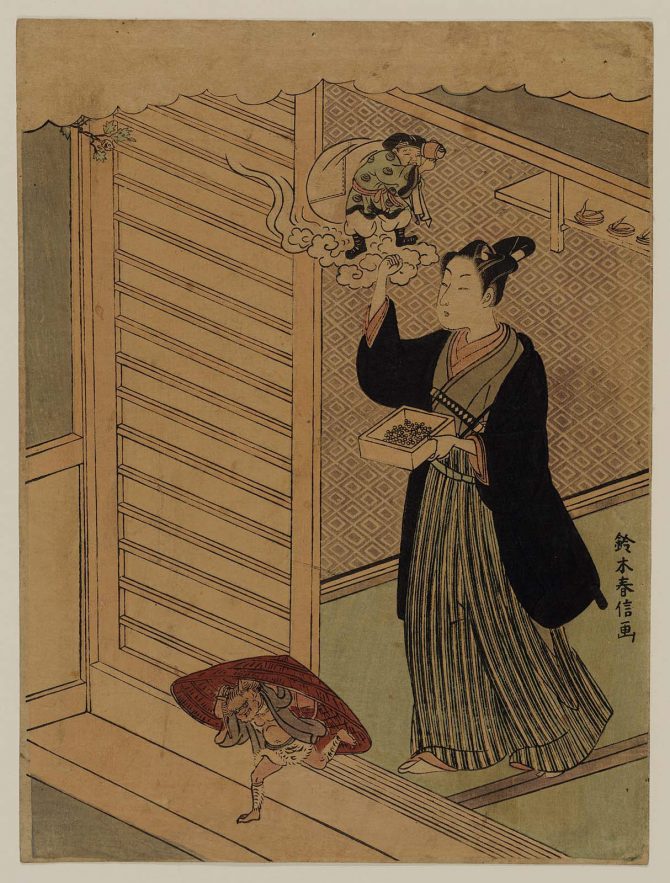The image depicts a vertical, framed illustration with a traditional Japanese or Chinese artistic style, combining pen and ink with some color highlights. Central to the artwork is a female figure with dark, pulled-back hair, clothed in a green-gray shirt, black overwrap, and long, striped pants. She stands barefoot, stepping out of a building. In her left hand, she holds a small box, while her right hand supports a small creature riding a cloud above her head. This creature, wearing a wide-brimmed, rose-brown hat, adds to the whimsical nature of the scene. Below her, another small figure resembling a toad, dressed in a bamboo hat and a diaper, is seen running away, carrying an air chest. The scene includes traditional Asian elements with some Chinese text on the right side, emphasizing cultural folklore. Splashes of green further accent the image, possibly indicating a sprig of greenery through a door on the left side.